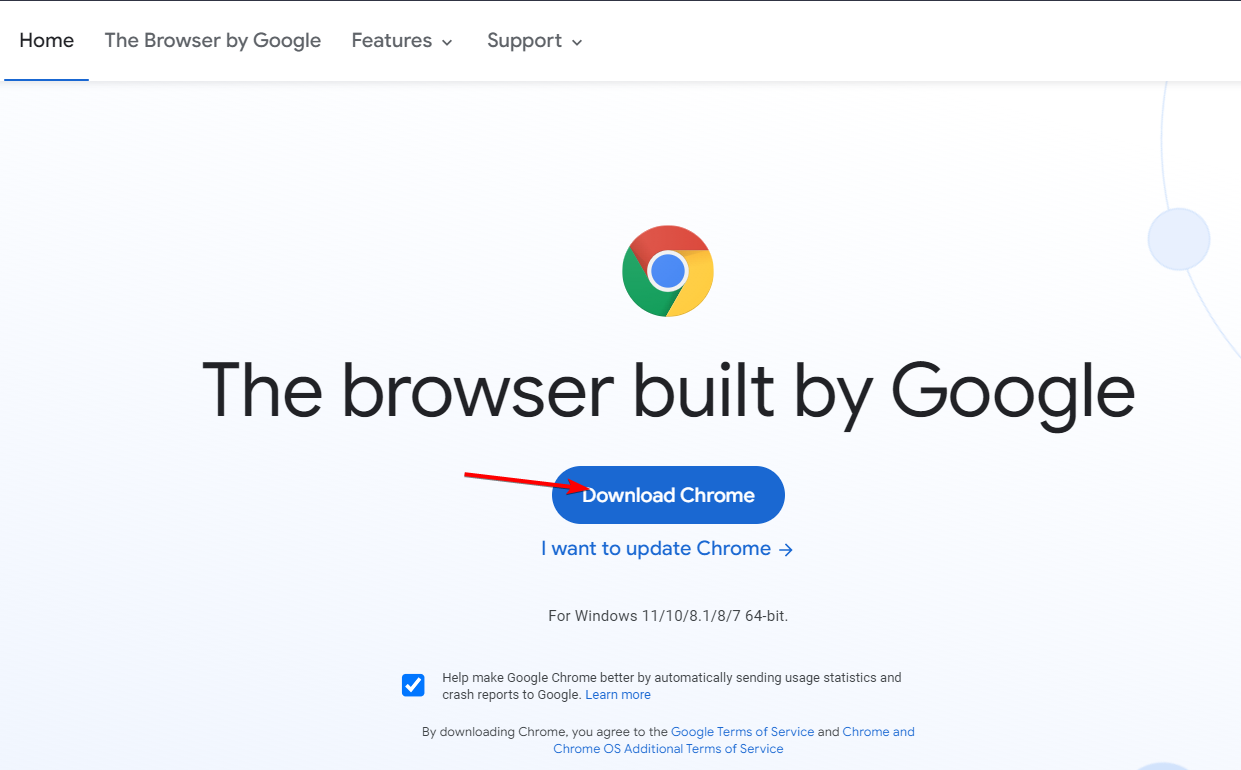This is a detailed screenshot of the Google Chrome browser download page on a digital device such as a tablet, desktop, phone, or laptop. 

At the top left corner, there is a bezel featuring a black line on the top and a faded gray line on the bottom, creating a shadow effect. On the far left of the interface, the word "Home" is prominently displayed in black with a dark blue underline. Beside it, the text "The Browser by Google" is visible. Adjacent to this, there's a tab labeled "Features" accompanied by a down arrow for additional options. Next to this tab is another tab titled "Support" also with a down arrow.

Centrally displayed is the Google Chrome logo, which is a circle divided into three curved sections: one-third red, one-third green, and one-third yellow, converging at a dark blue circle in the center. Below the logo, a bold black text reads "The browser built by Google."

Underneath this text, a red arrow points towards a prominent, dark blue, oval-shaped button centered on the screen. In this button, bold white text commands "Download Chrome." Below the button, a smaller blue text reads "I want to update Chrome" with a blue arrow pointing to the right.

Further down in a light blue section, it specifies the compatibility details: "For Windows 11/10/8.1/8/7," and mentions "64-bit" in black text.

A section below this includes a blue square with a white check mark and the text "Help make Google Chrome better by automatically sending usage statistics and crash reports to Google," alongside clickable blue text that says "Learn more."

Concluding the content, a new paragraph in black text states, "By downloading Chrome, you agree to the," followed by clickable blue text "Google Terms of Service," then in black, "and," and more clickable blue text reading "Chrome and Chrome OS Additional Terms of Service."